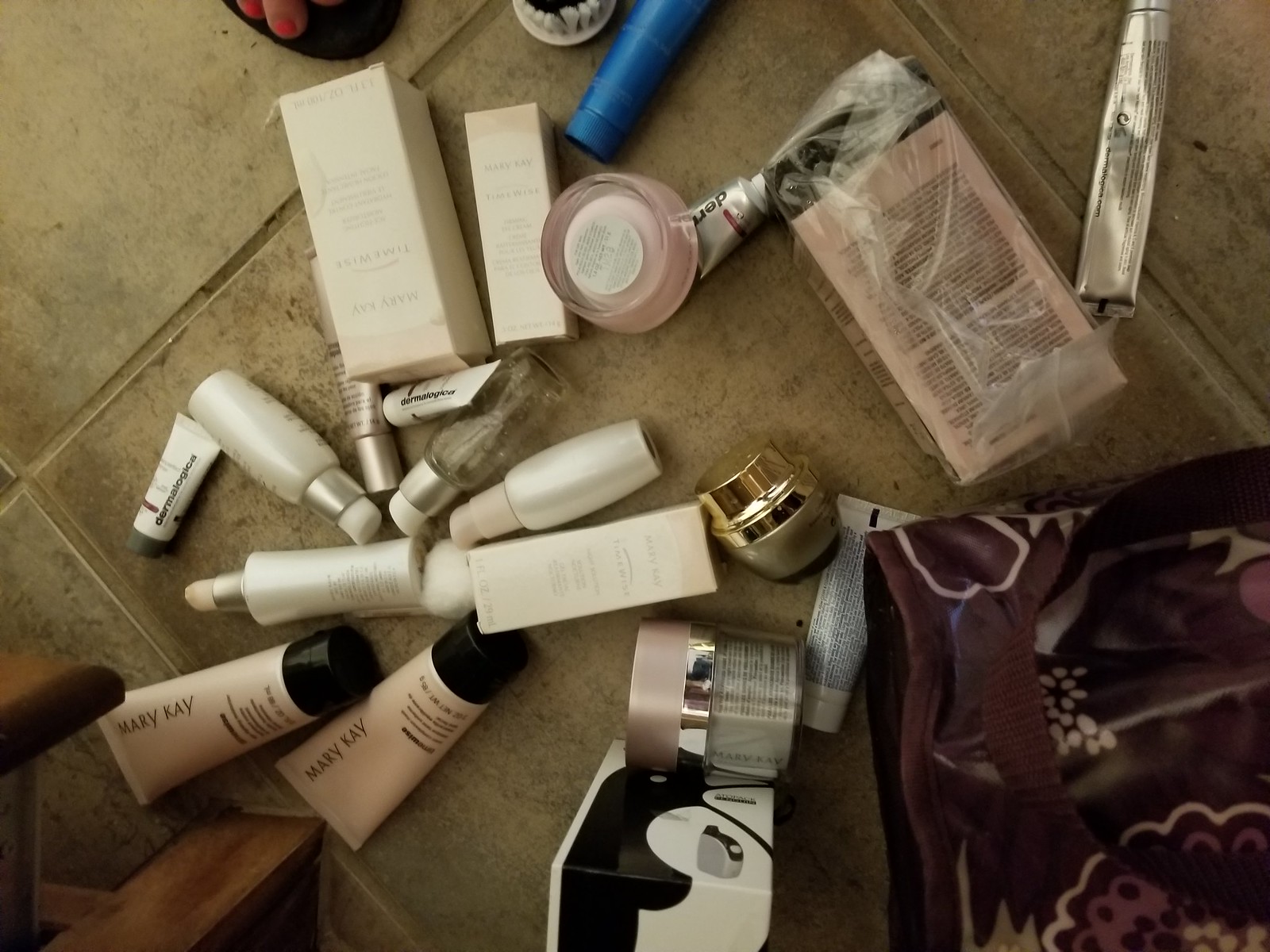This is a color photograph taken from above, capturing the scene of a countertop or tile floor. The rectangular image, slightly wider than it is tall, showcases a series of brownish tiles framed by grout lines. The perspective suggests the camera is positioned approximately two to three feet above the surface, zooming in closely to highlight about four tiles.

The tiles are scattered with various makeup items, indicating a sense of disarray. In the lower left corner, several Mary Kay tubes with black lids contain a pink substance. Adjacent to these, bottles with spray tops can be seen. A Mary Kay box, partially visible on the left side, adds to the clutter. 

Centrally placed within the frame are small cylindrical makeup holders in various colors and sizes, contributing to the mix of cosmetics. The upper right corner features packaging material, while a small silver tube occupies the far right corner. A blue cylindrical tube is noticeable towards the top center of the image.

A distinctive detail is the appearance of a toe in a sandal, peeking into the frame from the top left corner. In the bottom right, a portion of a package or a purse-like material is visible, suggesting that it may have been the source of the scattered items.